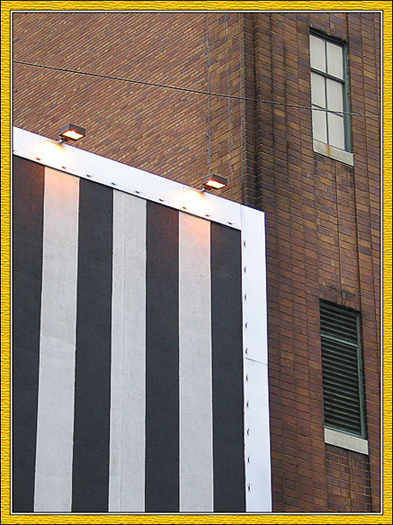This detailed portrait-style image showcases the side of a brick building with a vibrant outer yellow cartoon-like border. The brick building features red bricks arranged horizontally, with two slender rectangular windows. The top window is fitted with greyed-out panels, while the bottom window, adorned with green slits, resembles a wooden paneled window or metal grate that obscures visibility.

To the left of the brick building and occupying the left edge of the image lies another square structure, distinguishable by its black and white vertical stripes—three black and four white stripes—framed by a large white border. Two black lights hang from the top of this smaller building, casting a warm glow downward. The entire scene is framed by a thin yellow border, adding a whimsical touch to the photograph. The brick walls display a palette of brown, light yellow, and black, suggesting the image was captured during the day in an urban setting. No text is present within the image.